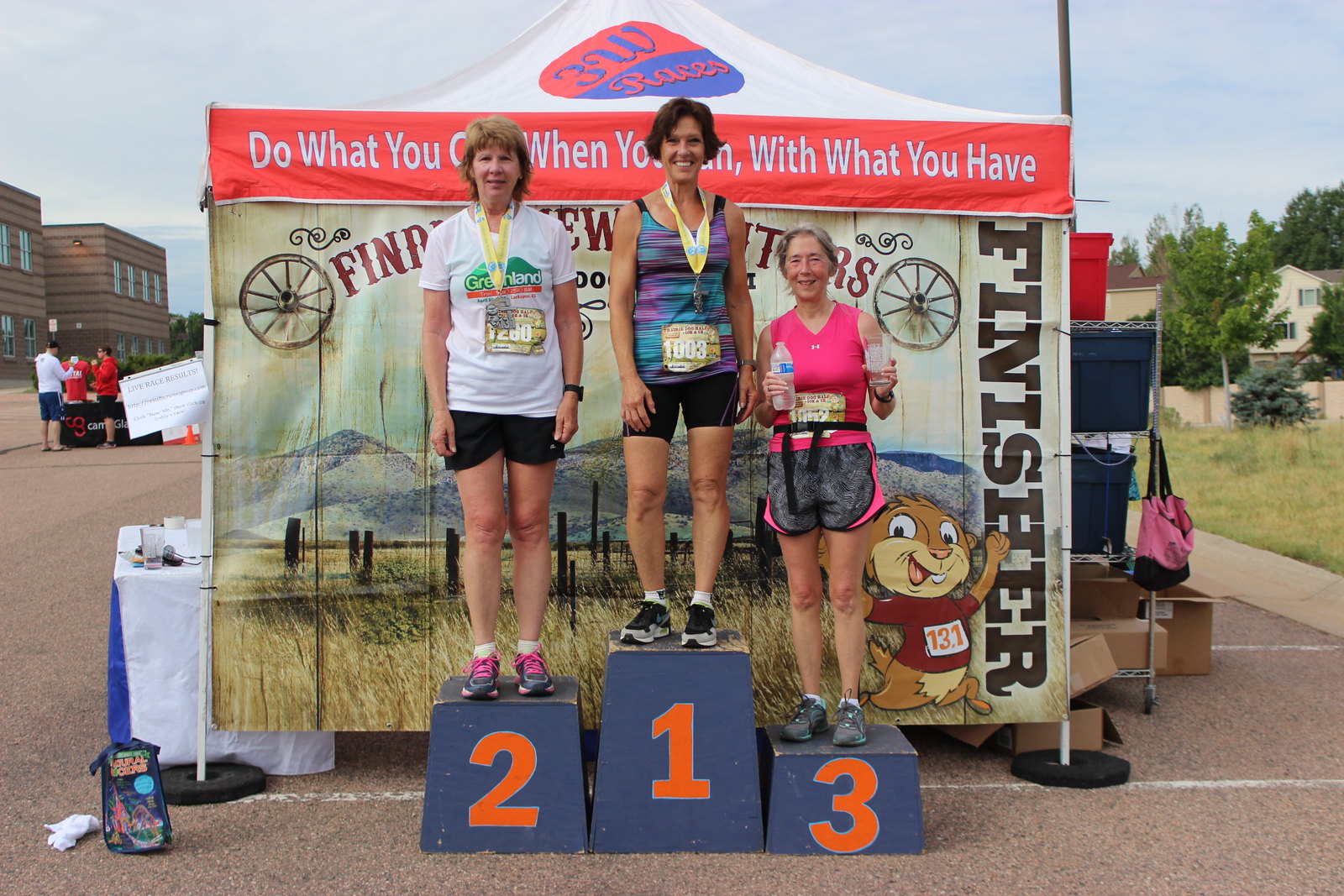This is a wide horizontal photograph capturing a post-race celebration with an outdoor makeshift winner's podium. The podium blocks are labeled with orange numbers: '1' in the center, '2' on the left, and '3' on the right. Standing atop these blocks are three women, all likely in their late 40s to 50s, each wearing shorts and short-sleeve tops while proudly displaying medals hanging from yellow lanyards around their necks.

The woman on the number 1 podium (center) is dressed in a pink and aqua tank top paired with black shorts. Her race number is '1003'. The runner on the number 2 podium (left) sports a white t-shirt adorned with an unclear image and dark shorts, bearing the race number '126080'. The woman on the number 3 podium (right) is clad in a pink tank top with pink and gray shorts and is holding a water bottle in her right hand and possibly a glass of water in her left.

Behind them stands a pop-up tent, partially shielding a sign featuring a chipmunk icon with a '13.1' inscription, indicating a half marathon event. The backdrop includes grassy areas dotted with trees and houses on the right, suggesting a slightly overcast sky with hints of blue peeking through, likely capturing a late afternoon scene. To the left in the background are three individuals - two in red tops and one in a white shirt - possibly race organizers or spectators.